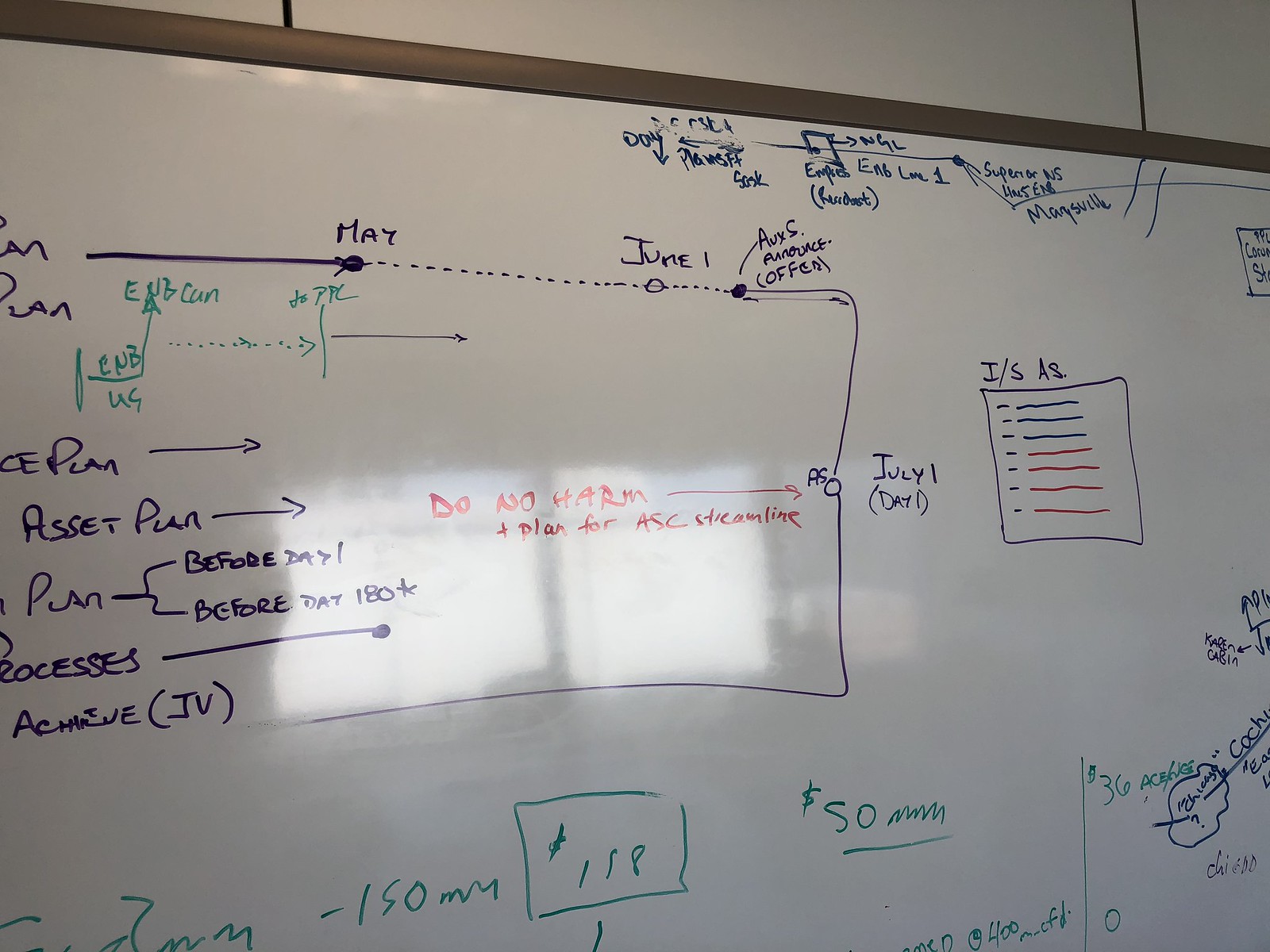The image depicts a whiteboard mounted on a white wall, framed by a thin brown wooden border at the top. The whiteboard is filled with various colorful writings including blue, purple, red, and green text. At the top middle, there is blue writing. Along the left edge, there's a vertically aligned column with partially visible names and words; this column is cut off on the left side. Near the top of the column, there's an arrow that points to a dot labeled "May," followed by a dotted line leading downwards to the label "June 1st." Further down, another dot with some text to its right appears. The line continues downward and curves to the left, ending at the bottom word in the left column.

In the middle section, written in red is the phrase "do not harm." Below this are some computations penned in green. On the bottom right, green writing overlays blue text. Toward the middle right, there's a square box marked with the notation "I/S, A.S." and contains dots and lines inside.

The board references an asset plan with multiple dates such as May, June 1st, July 1st, and July 11th. The left column includes terms like "process archive,” "plan before day one," and "before day 180." Some monetary amounts are also indicated in green. The setting of the whiteboard appears to be an office, possibly used by groups collaborating on an asset plan for a company. Additionally, the reflection of a computer can be seen on the whiteboard's surface.